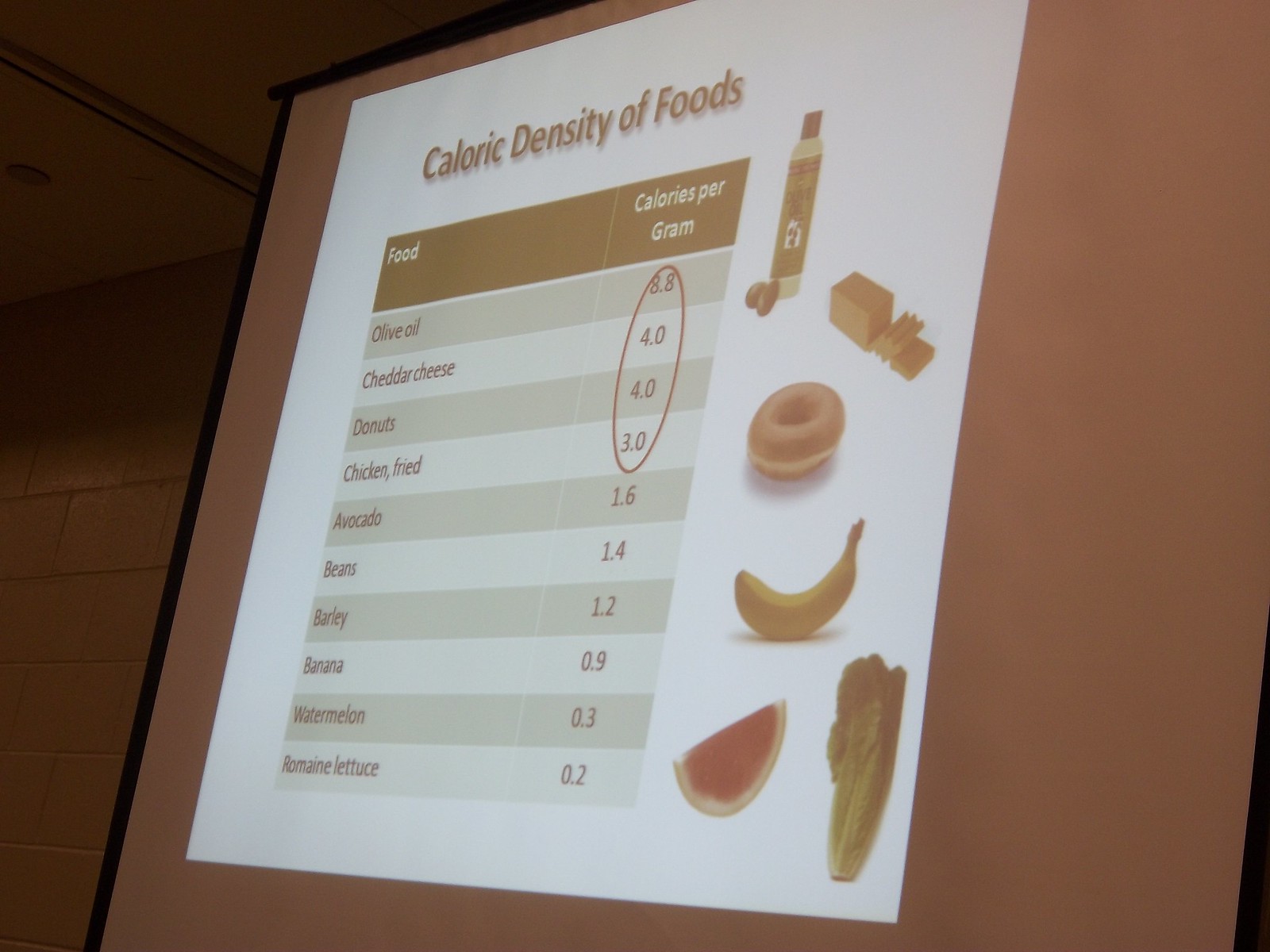This photograph captures an overhead projection screen displaying information about the caloric density of various foods. At the top, in a bold, dark font, is the title "Caloric Density of Foods." Below the title, the screen features a lighter-colored background with black text. Centered on this background is a black box with white text, listing two columns: one labeled "Food" and the other "Calories per Gram."

The list of foods and their corresponding caloric densities is presented in dark text against the white background as follows:

- Olive oil: 8.8 calories per gram
- Cheddar cheese: 4 calories per gram
- Donuts: 4 calories per gram
- Fried chicken: 3 calories per gram
- Avocado: 1.6 calories per gram
- Beans: 1.4 calories per gram
- Barley: 1.2 calories per gram
- Banana: 0.9 calories per gram
- Watermelon: 0.3 calories per gram
- Romaine lettuce: 0.2 calories per gram

On the other side of the image, there is an array of visual representations of these foods, including a bottle of olive oil, a donut, a banana, a slice of watermelon, and various vegetables. The detailed presentation provides a clear visual comparison of the caloric densities of these common foods.